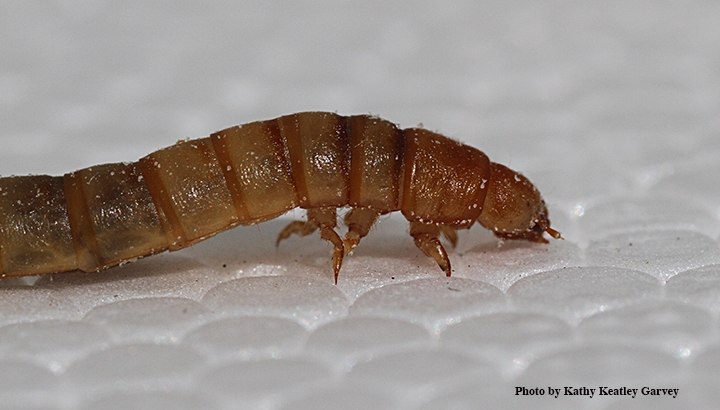This close-up image captures a detailed view of a mealworm positioned on a white, styrofoam-like surface. The mealworm, with its shiny, almost translucent brown body, appears wet and slightly damp. The creature's body is segmented, with visible divisions along its length—each a different shade of brown separated by darker bands. Only the front portion of its body has legs, consisting of small, delicate appendages that resemble the soft legs of a shrimp. Its rounded head, seen in a side profile, sports a small antenna and is tilted down towards the surface. Additional minute specks are visible on the mealworm, likely due to the magnification of the shot. The image also features a small, single-line watermark in black text at the bottom right corner, reading "photo by Kathy Keatley Garvey."